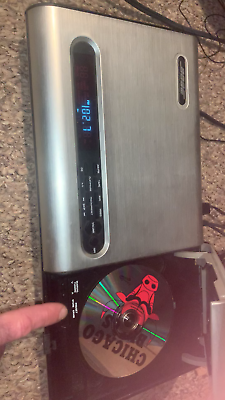The image shows a non-professional, tall photograph of an old, rectangular CD player, possibly by Bose, set in an indoor environment with visible wires in the background. The top half of the CD player features a silver control panel displaying a radio frequency of 102.7 and possibly the time. The bottom half reveals the CD tray with a disc labeled "Chicago Bulls," featuring an alien or skull-like figure. A finger is pointing at the exposed CD disc. The CD player and its technology appear outdated by modern standards. The image might originally have been taken in a landscape orientation but is shown rotated. The setting appears to be on a rug.